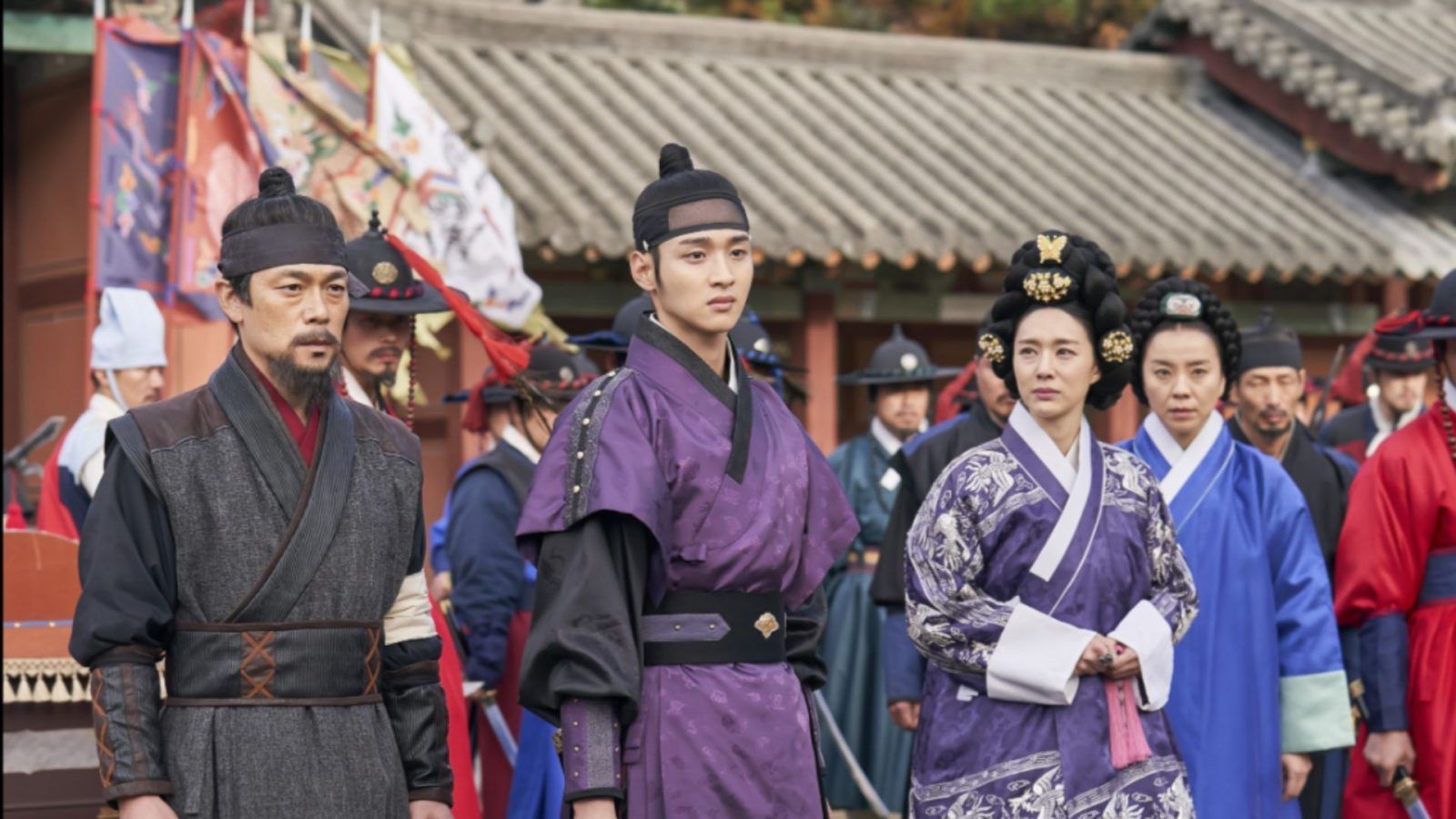The photograph, presumably taken in Japan or another part of the Far East, captures a group of four main individuals dressed in traditional Asian attire, possibly martial artists, standing outdoors in front of a traditional building with a gray roof. On the left, there's a man with a beard and mustache wearing a black stocking hat, black robe, and black belt. Next to him is another man in a purple robe with a black belt and cap. To his right stands a woman wearing a large black hat and a purple robe with white trim. Furthest to the right is another woman adorned in a light blue robe with white trim and a black hat. Both women have their hair pinned up. In the background, various flags are visible, along with homes and what appear to be soldiers wearing military hats, adding to the historical and cultural context of the image. The scene is brightly lit, emphasizing the clear details and vibrant colors of the robes and surroundings.